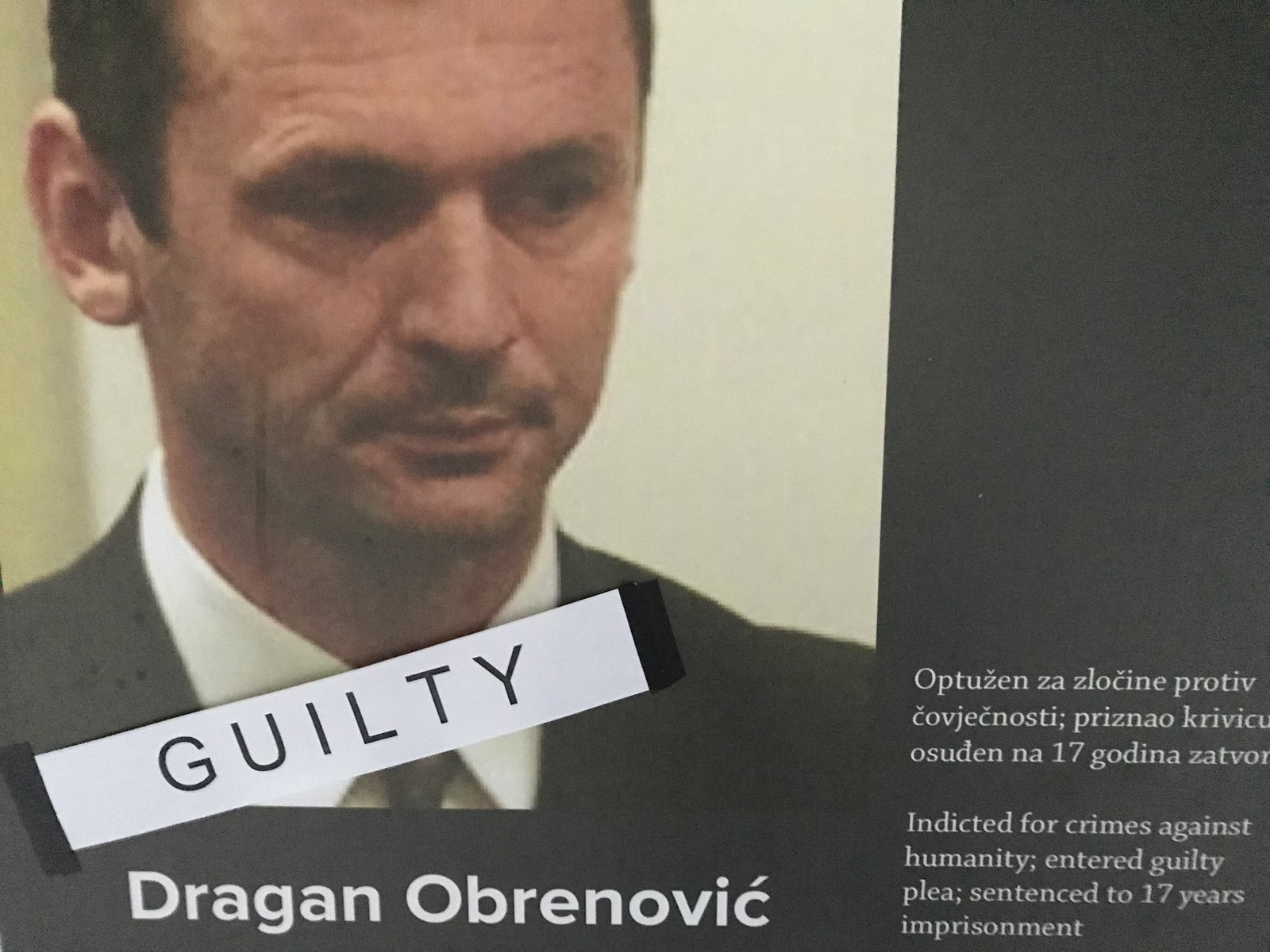The image portrays a head-and-shoulders photograph of Dragan Obrenovic, prominently occupying most of the left side of the frame and partially extending to the right. Dragan, a middle-aged man with short dark hair and a slight mustache, is dressed in a black suit, white shirt, and a darker tie. He bears deep wrinkles on his face and forehead. Superimposed over his neck and shoulders is a white rectangular label with the word "GUILTY" in bold, black uppercase letters. Below his image, his name, Dragan Obrenovic, is displayed. On the right side of the image, there is text in a foreign language, likely from Eastern Europe, accompanied by an English translation that reads: "Indicted for crimes against humanity, entered guilty plea, sentenced to 17 years imprisonment." The text is presented in white on a black background.